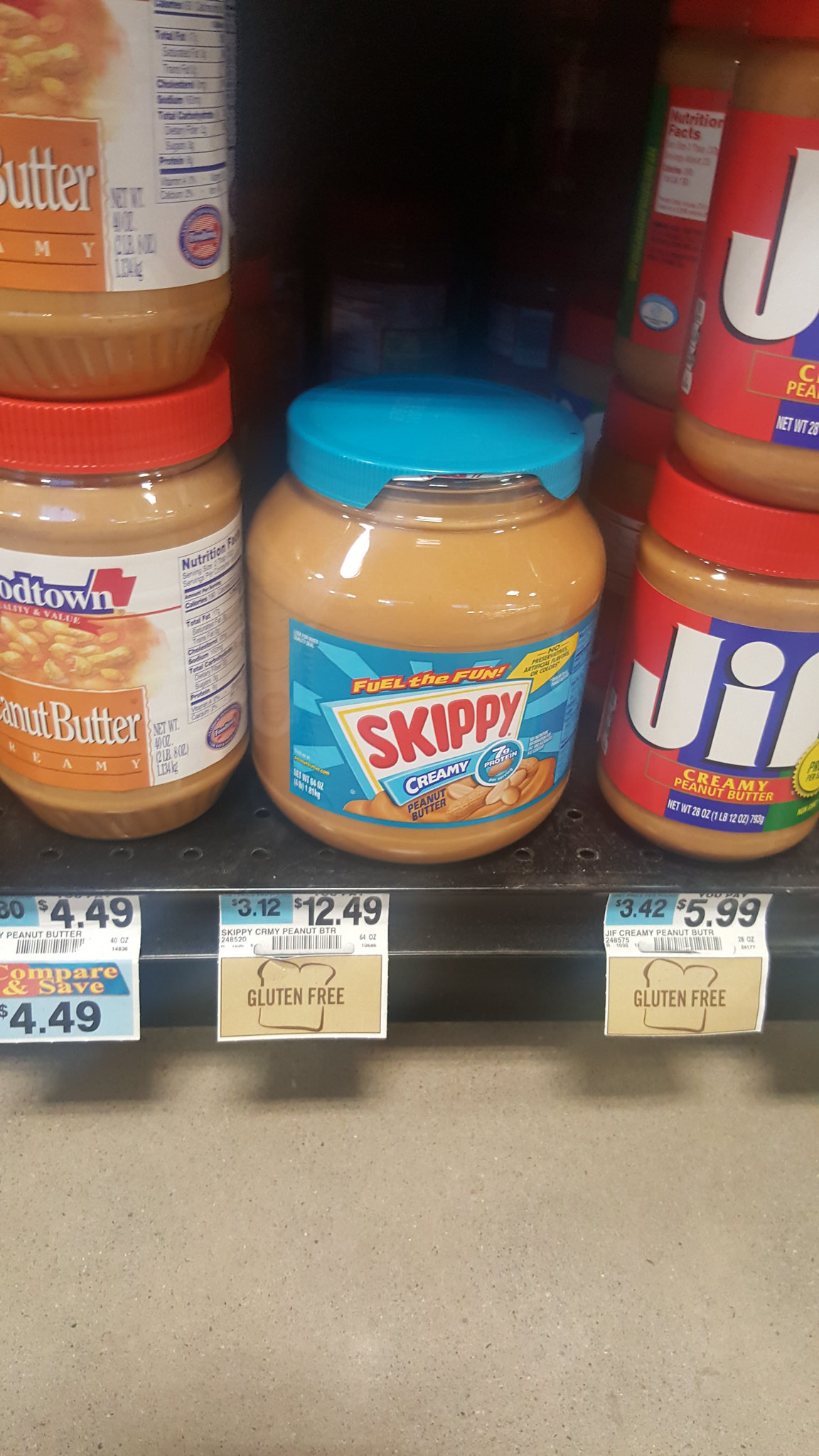Displayed in the image is a well-stocked grocery shelf showcasing various brands of peanut butter. The central focus is on a jar of Skippy Creamy Peanut Butter, distinctly marked by its blue lid, which is notably cracked with a small chunk of plastic missing. The Skippy jar flaunts its trademark blue label and is priced at $12.49, clearly marked as gluten-free. 

To the immediate right of the Skippy jar, there are neatly stacked plastic jars of Jif Peanut Butter, featuring their signature red caps and prominently labeled as gluten-free as well. The Jif jars are priced at $5.99 each. 

To the left of the Skippy jar is the Food Town brand peanut butter, housed in plastic jars with modest red lids. The Food Town peanut butter is the most economical choice on the shelf, priced at $4.49 per jar. Each product is displayed with its respective price tag, providing clear options for consumers.